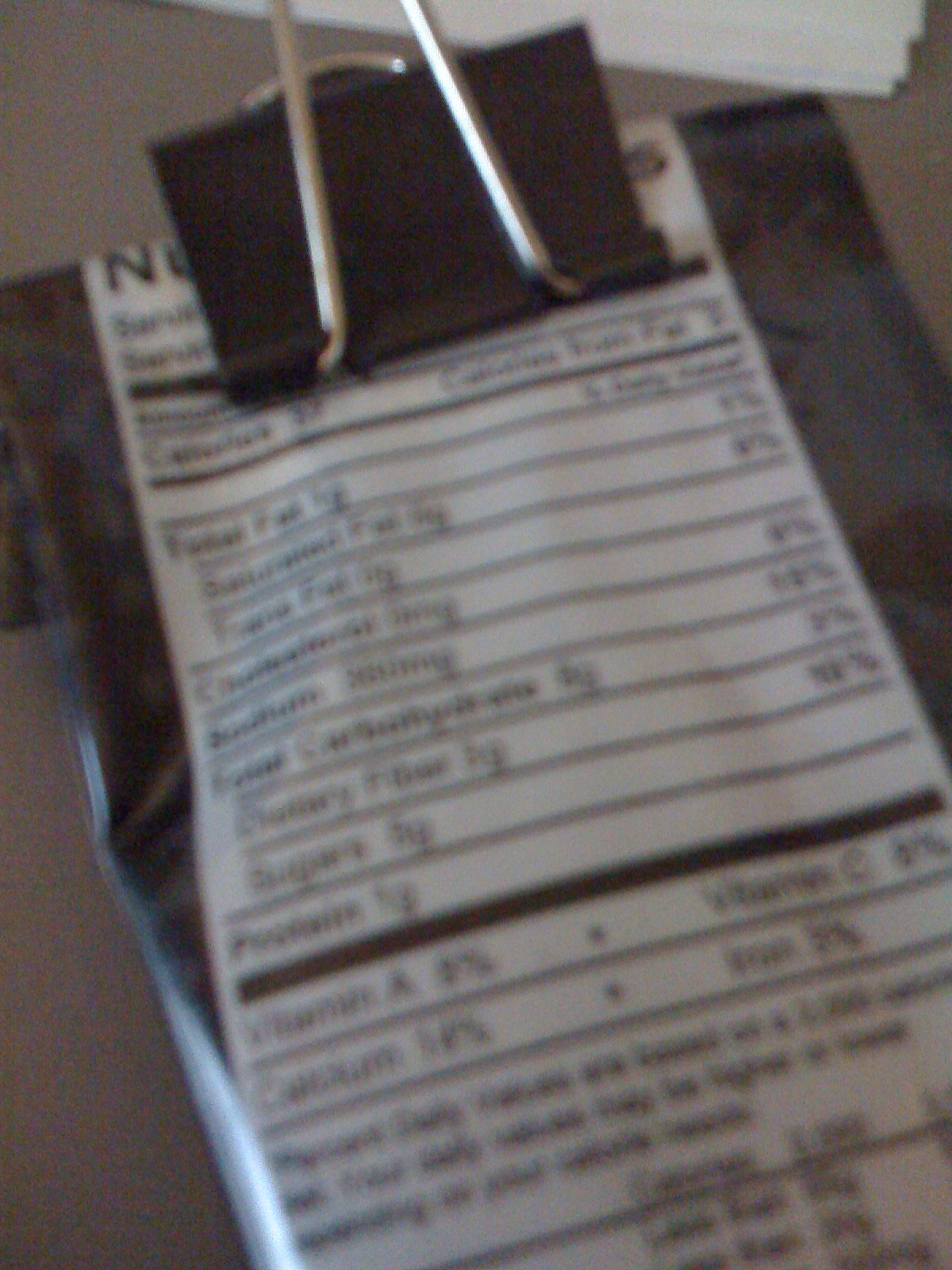In this image, a small, shiny black snack bag, resembling a foil-type material, is featured prominently. The bag is clamped at the top with a small black and silver clamp, which appears disproportionately large compared to the bag itself. The front of the bag displays a Nutrition Facts table with black text on a white background, although the image is so blurry that neither the lettering nor the numbers are legible. The bag is placed on a gray surface, likely a table or counter. In the background, there are three white sheets of paper stacked on top of each other, adding some context to the setting.